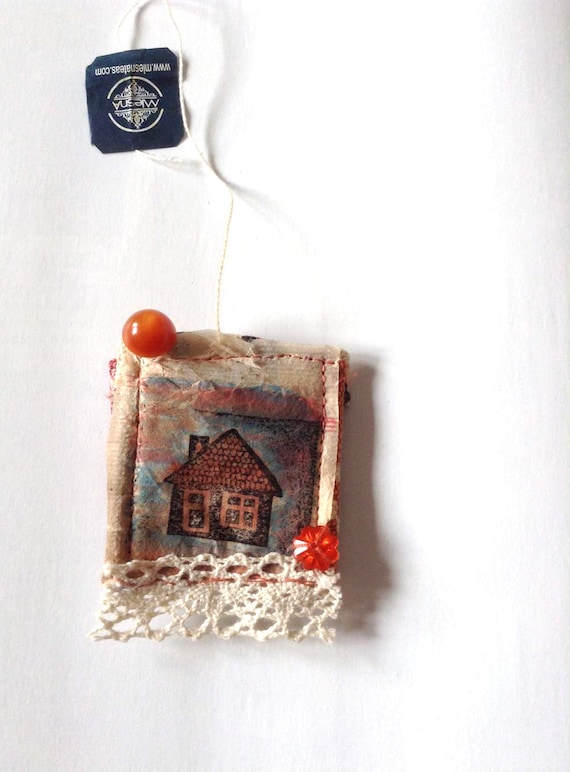The image features a vertically-oriented, rectangular photo set against a textured, predominantly white background with a bright white streak in the center resembling sunlight reflection. Centered within the image is a light brown teabag that appears old. Attached to the teabag by a thin white string is a small, navy blue square paper label positioned at the top left, adorned with an upside-down, white, swirly logo and some illegible text. The teabag itself displays the watercolor depiction of a simple house, characterized by blue siding and a pink roof with matching doors and windows. Surrounding the house are vibrant, watercolor hues of blue, purple, and red. The top left of the teabag features a coral, orangey-red bead or gem, while the bottom exhibits a lace-like cream-colored netting, accompanied by a small, flower-patterned bead on the bottom right corner.